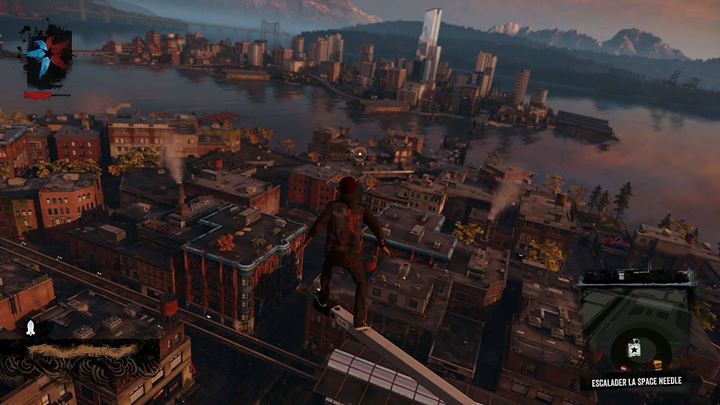This screenshot from a high-quality, three-dimensional video game shows an aerial view of a bustling cityscape. The scene is set as the sun begins to set, casting a pink and gray hue across a reflective body of water that divides two city sections. In the bottom right corner, the text "Escalada La Space Needle" suggests the game is either Spanish or set to the Spanish language. Above this text is a small icon, while a red-and-blue starfish-like icon with a half-filled progress bar appears in the top left corner. 

A human character, wearing a hoodie and black pants, balances precariously on a wooden beam extending from a high building, offering a dramatic viewpoint over the city below. The detailed cityscape features a mix of residential, commercial, and factory buildings. Prominent tall skyscrapers of silver, brown, and red are illuminated by the setting sun, further enhancing the scene's dynamic lighting. In the background, a bridge and a small island can be seen, with distant mountains framing the picturesque horizon.